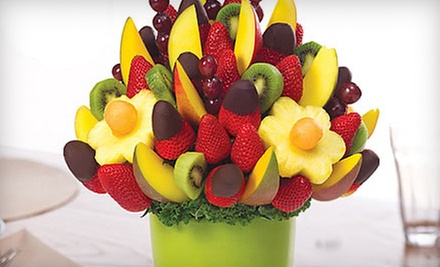The image depicts a vibrant and festive fruit bouquet arranged in a lime green base, resembling a flowering plant in full bloom. This delightful display of fruit is meticulously crafted to appear like a floral arrangement. It includes whole and chocolate-dipped strawberries, pineapples intricately cut into flower shapes with small cantaloupe or muskmelon centers, as well as slices of kiwi and possibly apples. Clusters of grapes are artfully positioned on sticks, adding to the bouquet's intricate design. The arrangement is situated on a table, with a blurred clear glass to the right and a place setting with a circular brown placemat or plate and a brown napkin to the left. Dark greenery peeks out from the top of the vibrant base, further enhancing the appearance of a lush, edible garden.